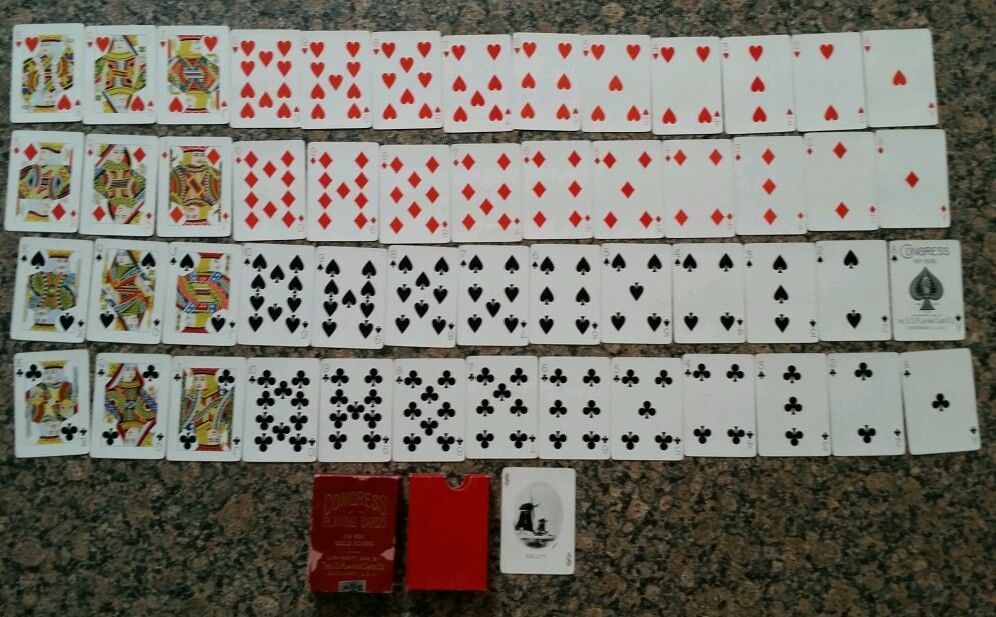In the image, a neatly arranged deck of playing cards is displayed horizontally on what appears to be a rough, textured floor. The floor's design mimics the appearance of dirt with a brown and black color palette, creating a rugged backdrop. 

The card arrangement begins with the top row featuring the Red Hearts suit, laid out sequentially from King, Queen, Jack, 10, 9, 8, 7, 6, 5, 4, 3, 2, to Ace, moving from left to right. Below the Hearts, the second row mirrors the first row with the Red Diamonds suit, also arranged from King to Ace in the same sequential order.

The third row, positioned centrally in the image, displays the Black Spades suit in the same sequential pattern from King to Ace. Notably, the Ace of Spades has a distinct design, bearing the word "Congress" and a special spade logo that differs from the traditional look of the other spades.

The fourth and final row, at the bottom, features the Black Clubs suit, again arranged from King to Ace. At the very bottom of the image, a red deck box is visible, showcasing the brand name "Congress" on its exterior.